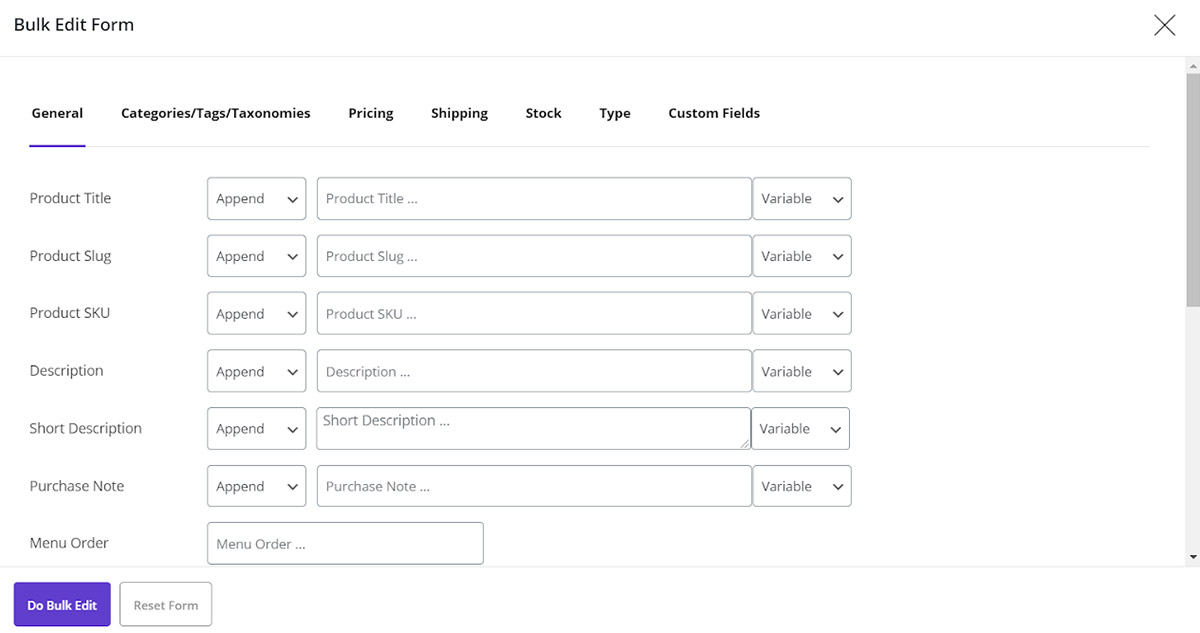### Caption:

The image showcases a form interface on a white background with black text. On the upper left, the label "BULT EDIT FORM" is prominently displayed. To the extreme right, there is a grey 'X' icon. Below this upper section, a grey horizontal bar spans the width of the form. Right beneath this bar, a series of categories and tags such as "GENERAL", "CATEGORIES", "TAGS", "TAXONOMIES", "PRICING", "SHIPPING", "STOCK", "TYPE", and "CUSTOMS" are listed in black text. The "GENERAL" category is highlighted in blue.

Further down on the left side, the form fields include "PRODUCT TITLE", "PRODUCT SLUG", "PRODUCT SKU", "DESCRIPTION", "SHORT DESCRIPTION", "PURCHASE NOTE", and "MENU ORDER". 

Each field offers a blue checkable box labeled "DO BULK EDIT" and a "RESET FORM" button next to it, presumably to clear input. Adjacent to these fields is a dropdown menu labeled "APPEND", and at the bottom, another labeled "ORDER MENU". 

Each text field, such as "PRODUCT TITLE", "PRODUCT SLUG", "PRODUCT SKU", "PRODUCT DESCRIPTION", "SHORT DESCRIPTION", and "PURCHASE NOTE" has an associated input area for user entry. Beside each field is a dropdown labeled "VARIABLE" that provides additional options.

A scrollbar on the right side signals the ability to navigate further down the form, with the top portion of the scrollbar being grey, indicating the current position at the top of the screen. This completes the overview of the form interface.